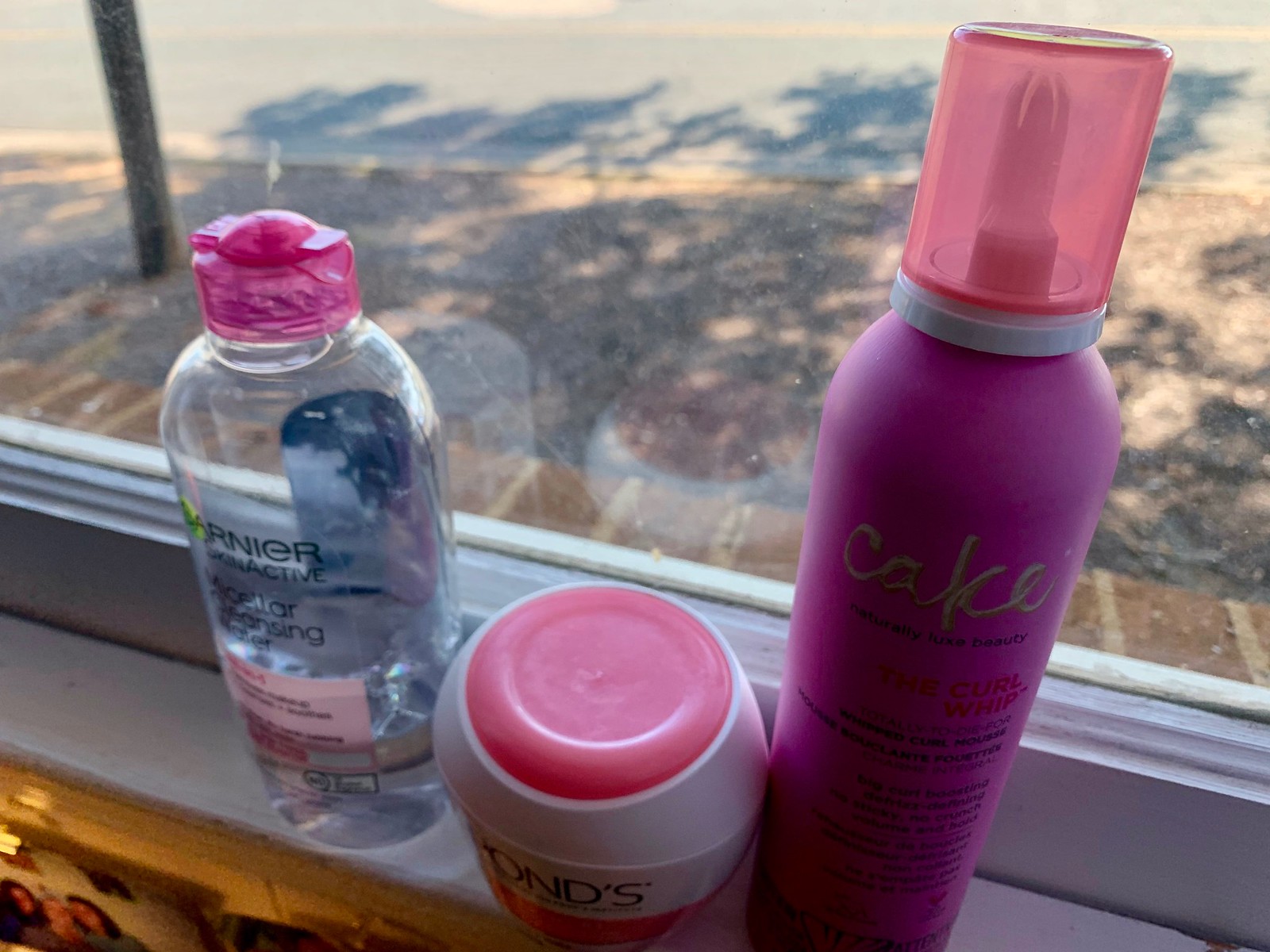In this detailed image, you are focusing on a windowsill. The window offers a clear view of the outdoors, where a sidewalk is visible. The glass of the window is also prominently featured. Positioned on the sill are three plastic containers, presumably personal care products.

The first container on the left is a clear plastic bottle labeled "Garnier." It contains a white liquid and has a pinkish-red cap. The second container is a small jar with a distinctive pink lid, identified as a POND'S product, spelled P-O-N-D-apostrophe-S. The third item is a purple, metallic, oval-shaped tube with a clear red cap, resembling a hair mousse dispenser.

Below the windowsill, there is a picture displaying a group of people. This image subtly adds a personal touch to the scene, indicating a possibly lived-in space with care products nearby.